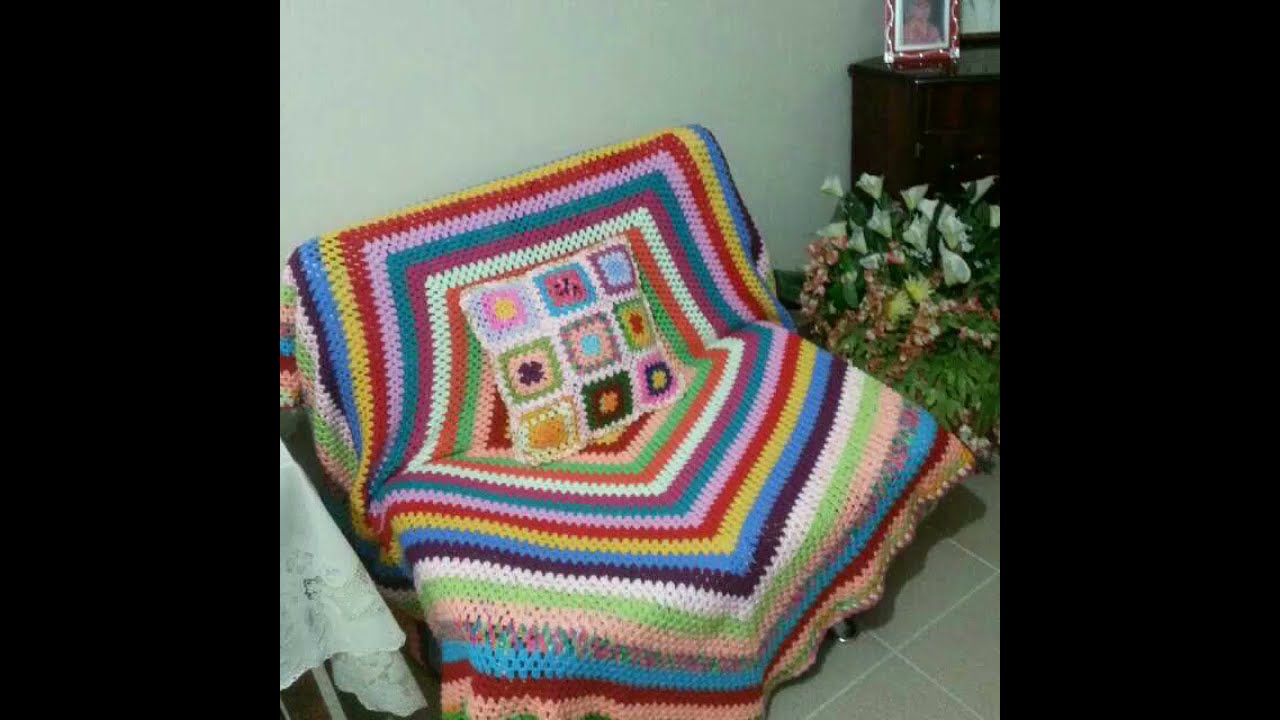In the center of this horizontally rectangular photograph, framed by large vertical black bars on the left and right, is a cozy, craft-themed scene within a room. Dominating the image is a large chair completely covered by an intricately crocheted, multicolored blanket, showcasing a variety of geometric patterns. At the core of the blanket is a pentagonal structure that extends outward in layers of vivid colors, including shades of pink, white, green, blue, several purples, yellow, as well as teal, magenta, orange, and peach. Central to the blanket's design is what appears to be a square pillow or part of the blanket itself, consisting of nine smaller squares each featuring distinct crocheted patterns and colors.

The background features an off-white wall, creating a clean backdrop along with a tan tiled floor beneath. To the right of the chair, there's a large potted plant displaying white, orange, yellow, and pink flowers, adding a natural touch to the scene. Also on the right, partially visible, is a chest of drawers topped with a framed picture, further enhancing the homey ambiance. On the left of the chair stands a smaller table adorned with a delicate lace white tablecloth, contributing to the room’s quaint and inviting feel.